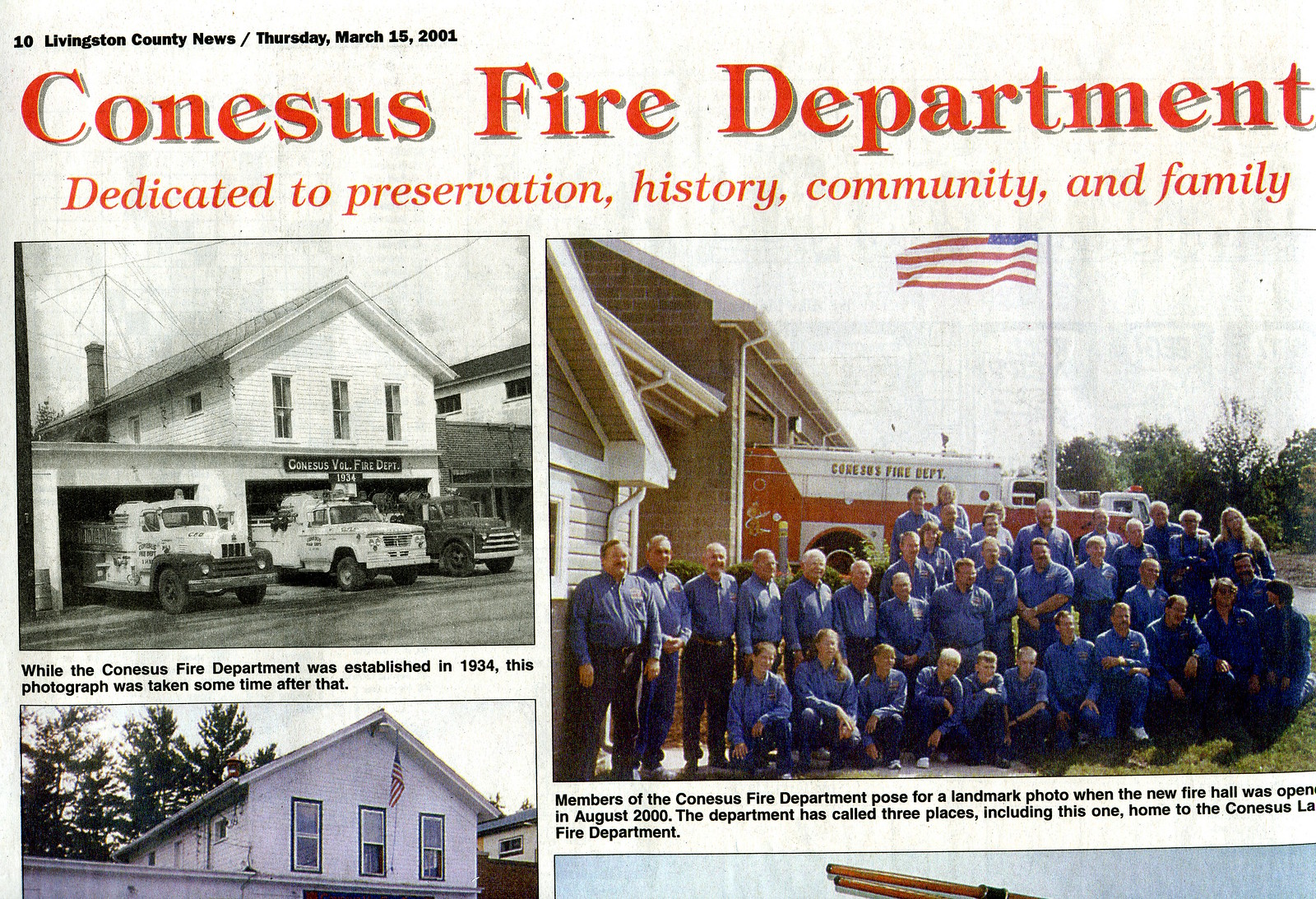The image is a detailed layout from a newspaper article, prominently titled "Consensus Fire Department" in red at the top. Below, there is a caption, "dedicated to preservation, history, community, and family" in black. The article, from the Livingston Community News, dated Thursday, March 15th, 2021, contains two central photographs comparing past and present. 

On the left, a black-and-white photo depicts the Consensus Fire Department as it was in 1934, showing a historic building with a group of firefighters. To the right, a modern color photograph captures the same fire department in the year 2000, with approximately 20 members in blue shirts and black pants, standing in front of a red and white fire truck, accompanied by an American flag. In the background, there's a white building with trees. The text below the modern photo notes that the firefighters posed for this landmark photo when the new hall opened in August 2000. The fire department has occupied three different locations over the years, including this new hall.

The overall presentation resembles a magazine or pamphlet dedicated to highlighting the enduring legacy and evolution of the Consensus Fire Department within the community.